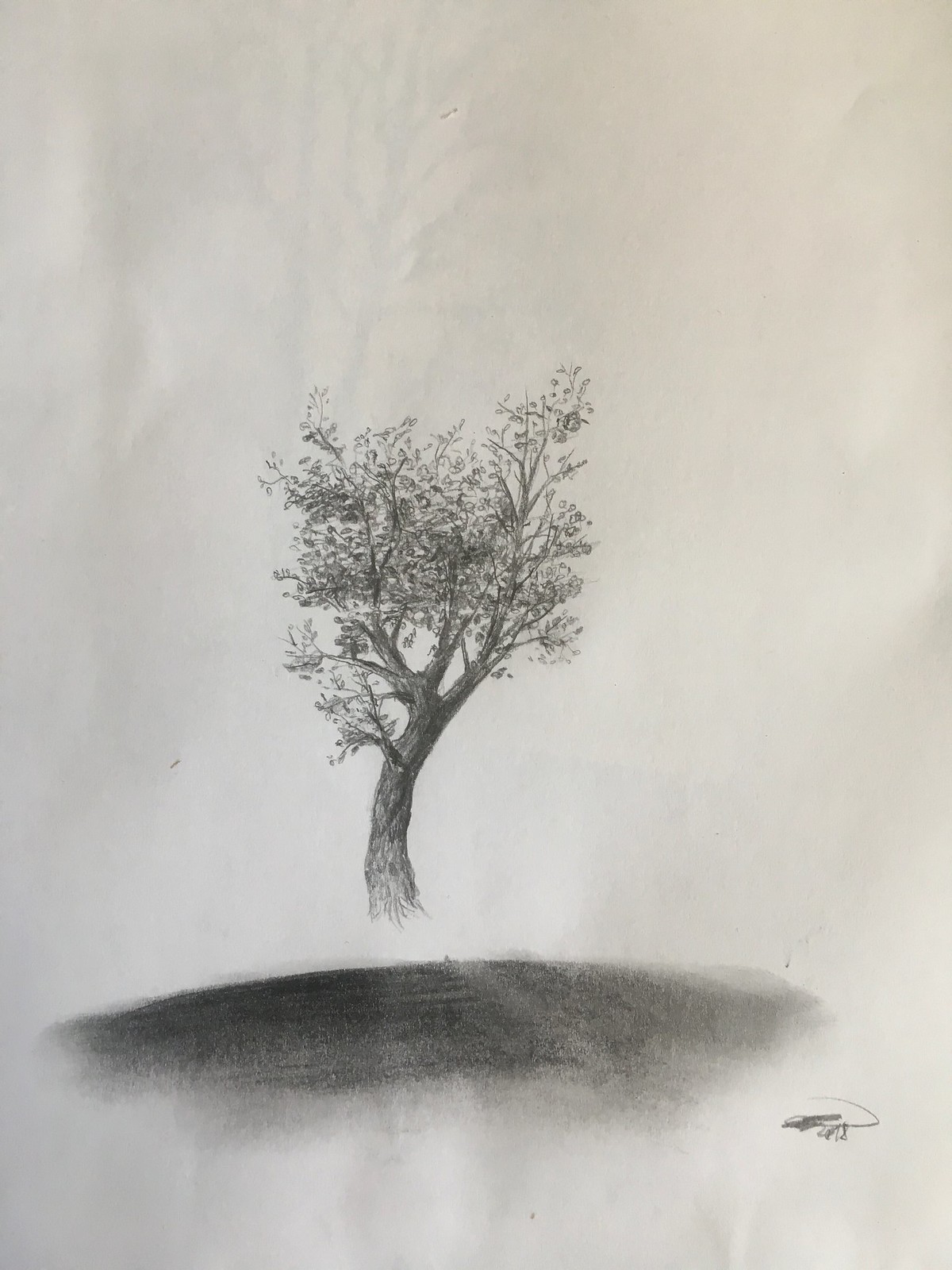This photograph captures a detailed drawing on a wrinkled white sheet of paper, possibly from a sketchbook or newsprint. The drawing, created with a sketch pencil or charcoal, primarily features a meticulously detailed tree with visible bark textures and abundant foliage, which may include flowers or fruit resembling pears or apples at the top. The tree intriguingly hovers above a nondescript ground, which is represented by a large, dark, smudged area in the foreground. The smudging appears to have been done with a thumb, giving the ground an indistinct, fuzzy effect. The lower right corner of the paper contains a small, scribbled signature, indicating the artist's mark without seeking notable recognition. The upper portion of the page remains blank, lending contrast to the densely detailed tree and adding to the surreal, enchanting quality of the drawing.